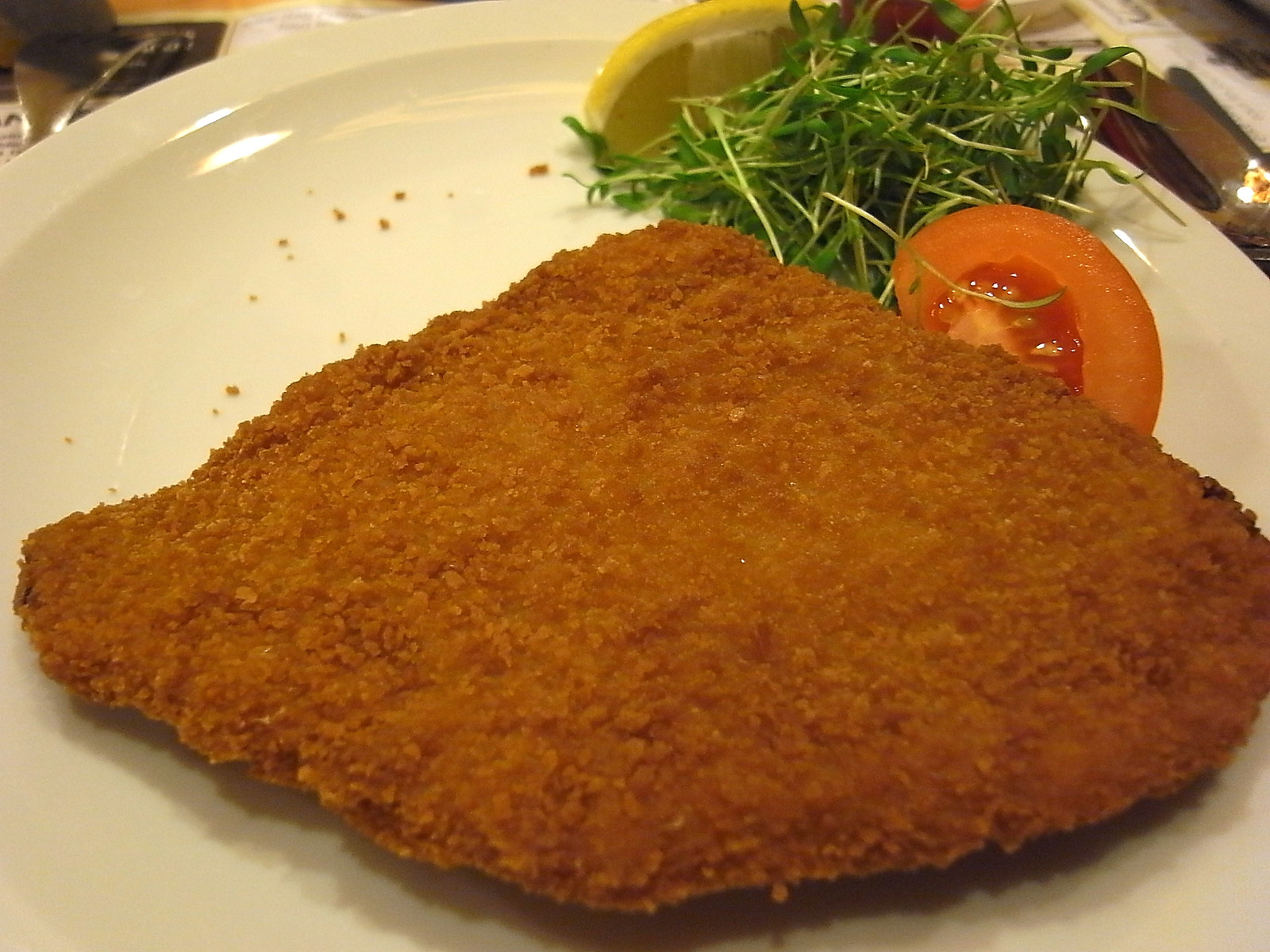The photo captures a simple and appetizing meal served on a white dinner plate. At the center, there's a large, breaded, and fried piece of meat, possibly chicken or fish, shaped like a thick diamond and occupying most of the plate. The fried meat left a few crumbs scattered around its edge. Garnishing the plate are a wedge of lime and a slice of beefsteak tomato, with sprigs of micro cilantro adding a touch of green between them. Additionally, there seems to be a hint of Brussels sprouts on the side. The setting appears to be indoors, accompanied by subtle details like a small candle on the right side, part of a spoon or fork, and possibly a menu in the top left corner, suggesting a dining experience.